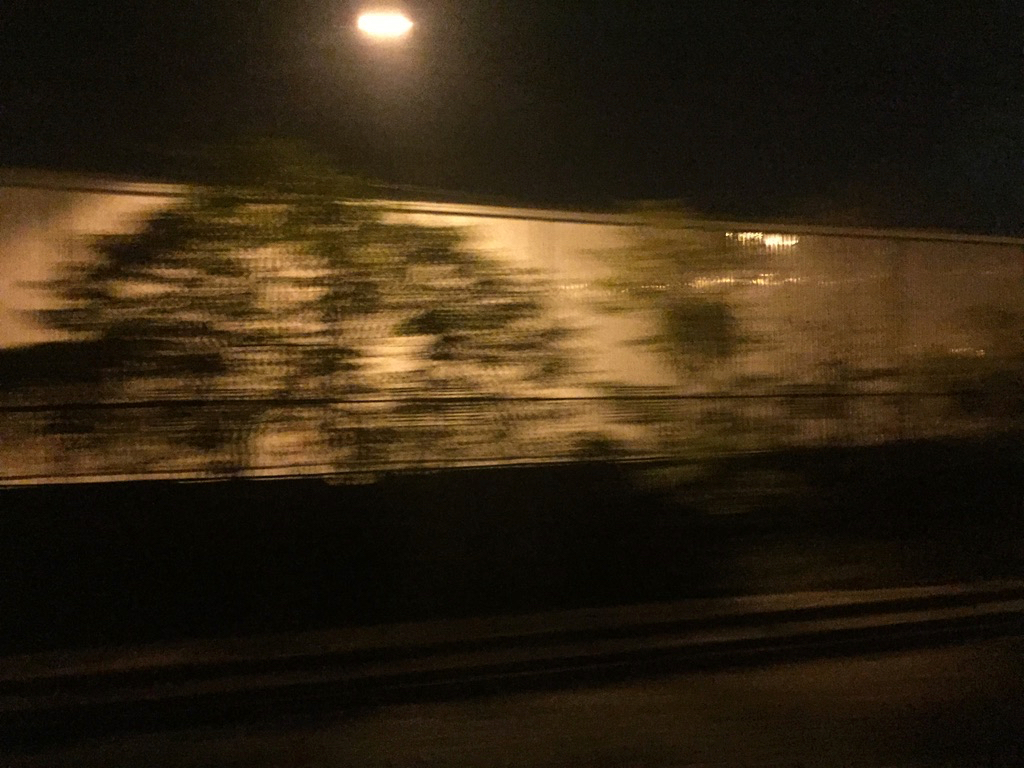A captivating nighttime photograph captures an urban scene bathed in the soft glow of a streetlamp. Positioned slightly to the left at the top of the image, the streetlamp emits a bright yellow light, casting a mixture of yellow and white illumination downwards. In the center of the frame, a white wall stretches horizontally from left to right, partially obscured by a row of slender, green trees. These trees appear to be in motion, lending a blurred, ethereal quality to the image. The bottom right corner hints at the presence of a street and possibly a sidewalk, though these areas are shrouded in near-total darkness. The wall also displays a faint yellow reflection in the middle, adding to the scene's mysterious ambiance.